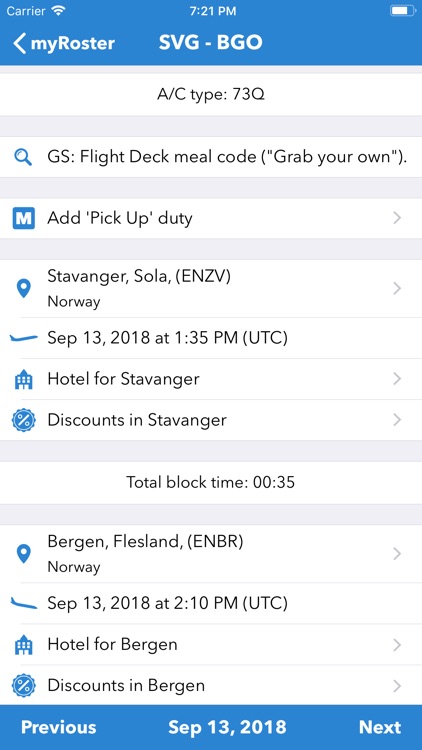A detailed screenshot of an airline roster displayed on a monitor. The screen header reads "My Roster," followed by details of a flight: "SVG-BGO." The flight section provides information including "AC Type: 73Q," "GS," and "Flight Deck Meal Code: Grab Your Own." Additional options on the screen include "Add Pickup Duty."

The itinerary for the day is detailed as follows: 
- "Stavanger Sola (ENZV), Norway - September 13, 2018, at 1:30 PM UTC," along with links for "Hotel for Stavanger" and "Discounts in Stavanger."
- "Total Block Time: 35 minutes."
- "Bergen Flesland (ENBR), Norway - September 13, 2018, at 2:10 PM UTC," alongside "Hotel for Bergen" and "Discounts in Bergen."

At the bottom of the screen, there is a blue navigation bar with "Previous" and "Next" in white text, flanking the date "September 13, 2018."